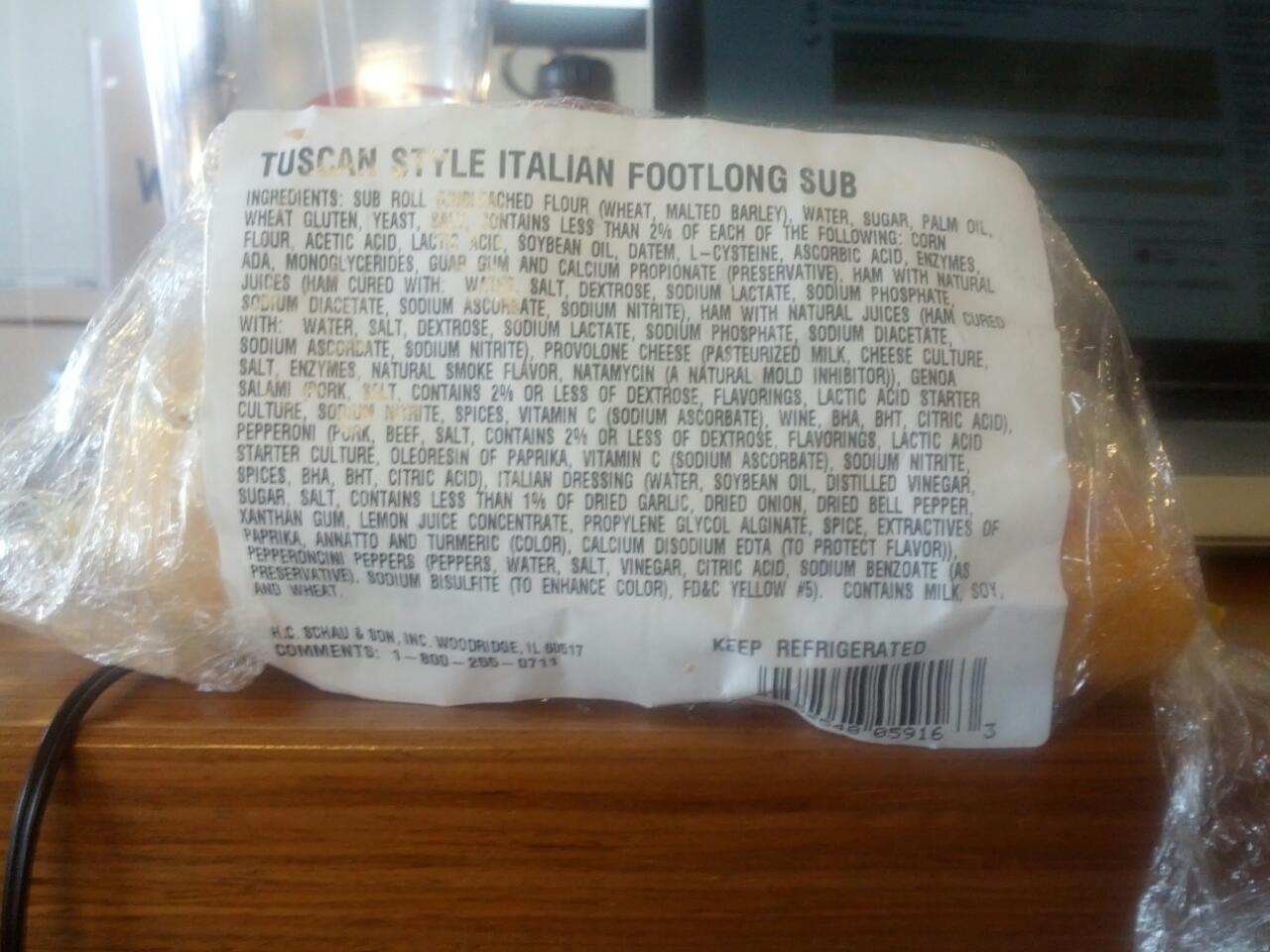In the center of the image, a sloppily-wrapped Tuscan Style Italian Footlong Sub, encased in a clear plastic cellophane bag, sits prominently on a wooden table. The packaging allows visibility of the bread at both ends, with a white paper label displaying the sub's name in black letters. The label also lists an extensive range of ingredients, including both natural components like flour, wheat, malted barley, water, sugar, and salt, and numerous chemicals. At the bottom right corner of the label, it advises to "keep refrigerated" and includes a barcode. Additional label details in the bottom left corner mention "Casey, Scholl and Son, Incorporated Woodstock, Illinois," along with a customer service number. Behind the sub, a black cord lays across the table's surface, trailing off the edge; it's connected to an unseen device—possibly a blender. The background reveals a kitchen setting, featuring a countertop and what appears to be an oven or microwave in the distance, partially obscured by shadows. A water bottle with a black lid and a bag potentially filled with goldfish crackers or an orange image also rest behind the sub, adding to the scene's cluttered, everyday atmosphere.